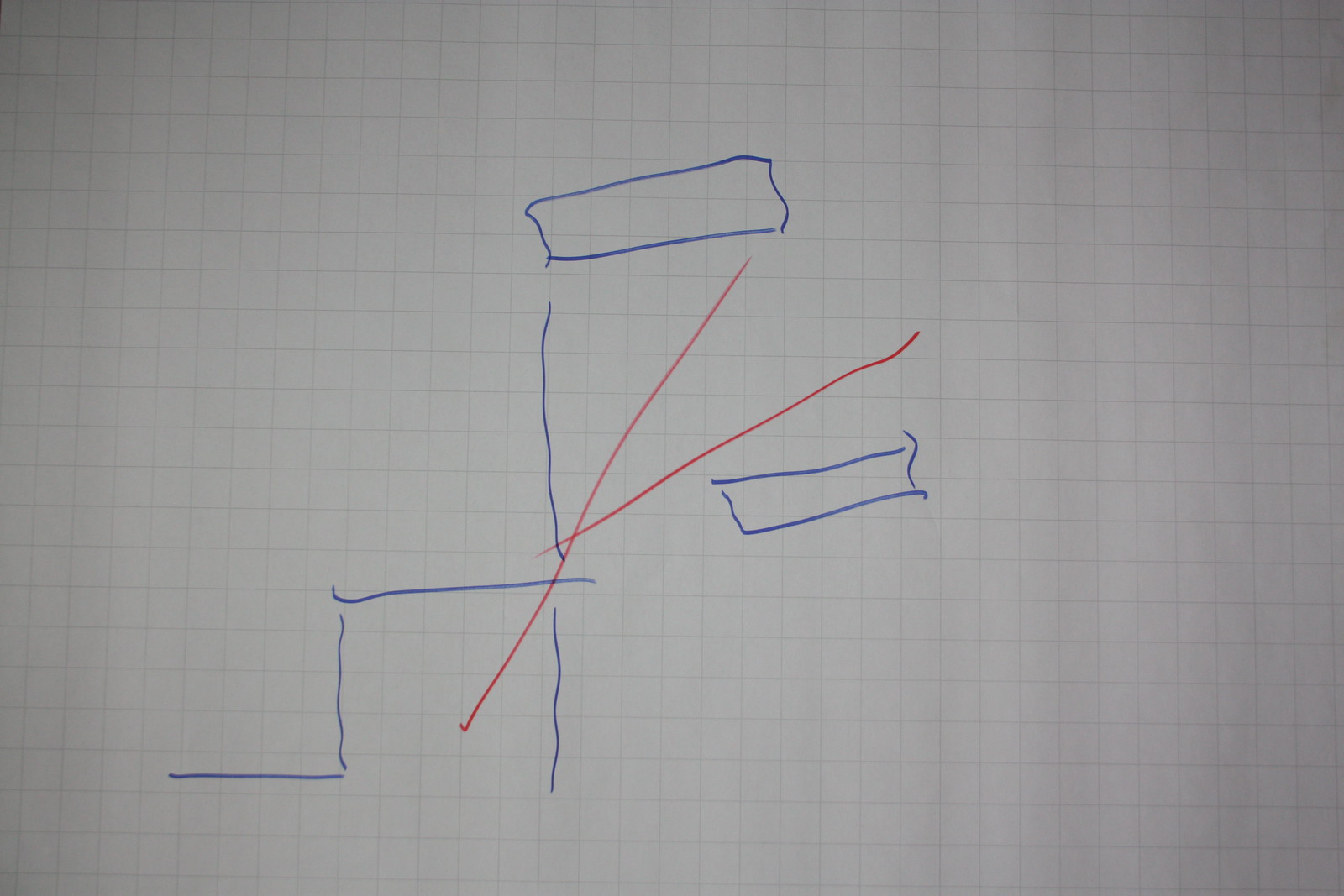This image captures a drawing made on a white, slightly rumpled sheet of paper. The drawing consists of blue and red ink, depicting a series of structured blue shapes that initially resemble stairs. The blue shapes include prominent rectangles, one positioned at the top and another beneath it. Overlaying these blue shapes are two intersecting red lines, forming a cross at the center. The photograph appears to be taken in dim lighting, casting shadowy outlines and soft shadows around the paper. The overall scene is minimalistic, focused solely on this intricate, yet ambiguous, doodle.